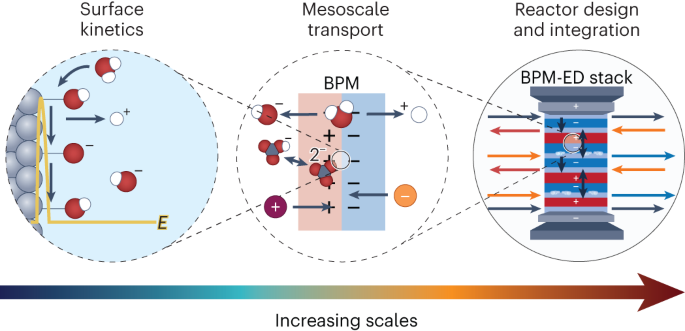This scientific illustration diagram depicts a multi-scale process divided into three interconnected sections. On the left, the illustration labeled "Surface Kinetics" shows molecules, specifically water molecules, dissociating and interacting, represented by red, blue, and white bubbles. Below this, a circle visually encapsulates these molecular actions. This circle flows into the next part labeled "Mesoscale Transport," where the same bubbles are shown moving within a different context, illustrating the transport stage within the process. The third section is "Reactor Design and Integration," featuring a detailed BPM-ED stack diagram, which likely represents a cylindrical reactor system with arrows indicating the dynamic movement of the molecules inside. Spanning from left to right beneath all these sections is a large arrow labeled "Increasing Scales," transitioning from cool to hot colors, symbolizing the progressively larger and more complex scales of the process from surface interactions to full system integration.